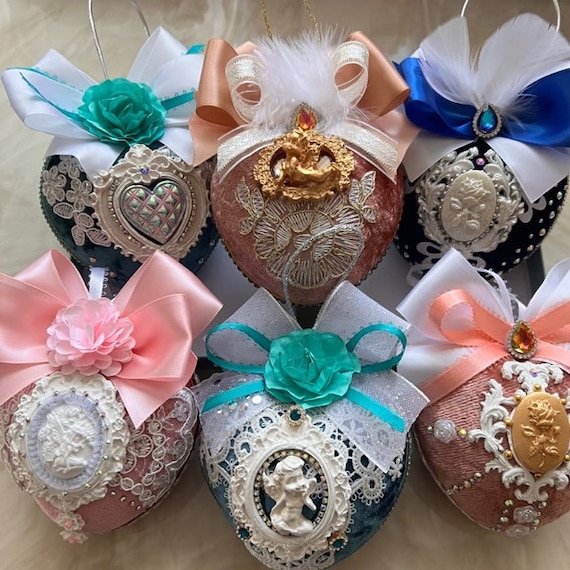The image depicts a set of six elaborately ornate decorations, likely intended as Christmas ornaments. Each ornament is a plush, heart-shaped piece featuring intricate appliqué or embroidered designs, including Victorian-inspired ivory emblems, flowers, and even faces. These decorations are adorned with a mix of pink and blue ribbons, some interspersed with white feathers and small gemstones, adding to their festive allure. Notably, each piece has a fabric loop at the top, indicating that they are meant to be hung, possibly on a Christmas tree. The ornaments vary in color, comprising pink, light blue, dark blue, and coral hues. The detailed craftsmanship suggests they were handmade with great care and an eye for elaborate detail, lending an air of grandiosity and charm suitable for festive or romantic occasions.